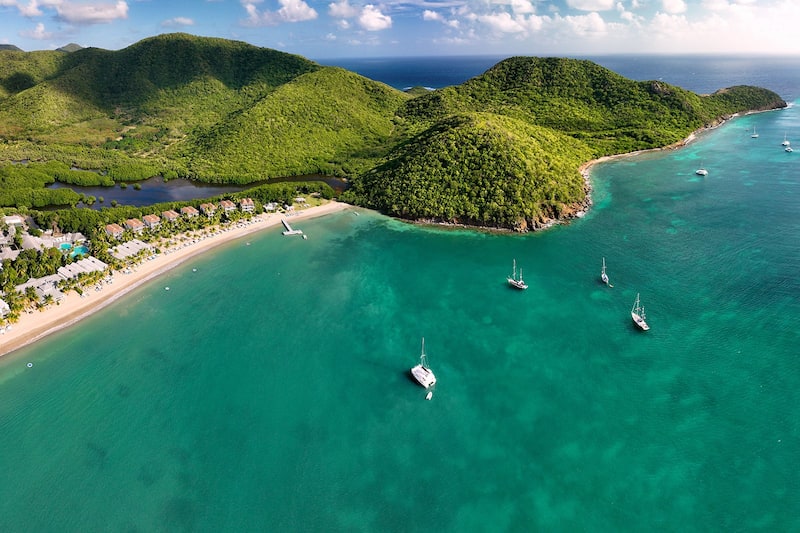This stunning aerial photograph captures a vibrant coastal landscape bathed in natural daylight. Taken from a high vantage point, likely using a drone, the image showcases a panoramic view of a lush, green island surrounded by the rich, teal-colored ocean. The island itself is adorned with verdant hills densely covered in trees, creating a striking natural tapestry that draws the eye. 

In the foreground to the left, there is a pristine white beach lined with what appears to be apartments or hotels, hinting at a popular vacation spot. A small pier juts out into the crystal-clear tropical waters, suggesting leisure activities and holidaymakers enjoying the serene environment. The water is so clear that the boats floating on it cast distinct, sharp shadows, enhancing the scene's tranquil, idyllic quality. Among these vessels, one particularly larger boat stands out, possibly a small yacht, adding a touch of luxury to the view.

The upper portion of the image features a bright blue sky streaked with wispy white clouds, indicating a perfect, sunny day. The clarity and brightness of the entire scene emphasize the vivid colors and details, making this photograph a breathtaking visual escape into a serene coastal paradise.